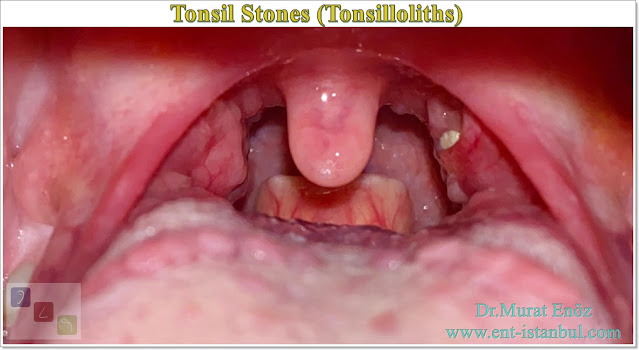The image is a detailed, close-up view of the inside of a person's mouth, focusing on the throat area. At the top of the rectangular image, in white letters, is the title "Tonsil Stones" with "Tonsilloliths" in parentheses. The scene predominantly features shades of pink, with some white, gray, and red. The visible anatomy includes the roof of the mouth, the uvula hanging from the top, the back of the tongue, and the tonsils. Notably, there is a white discoloration, resembling a tooth, on the right tonsil, indicating the presence of tonsil stones. The entire image suggests a medical context. At the bottom right, teal-colored text displays the website "www.ent-istanbul.com" and mentions "Dr. Murat Enos." Additionally, there is a faint logo at the bottom left corner.